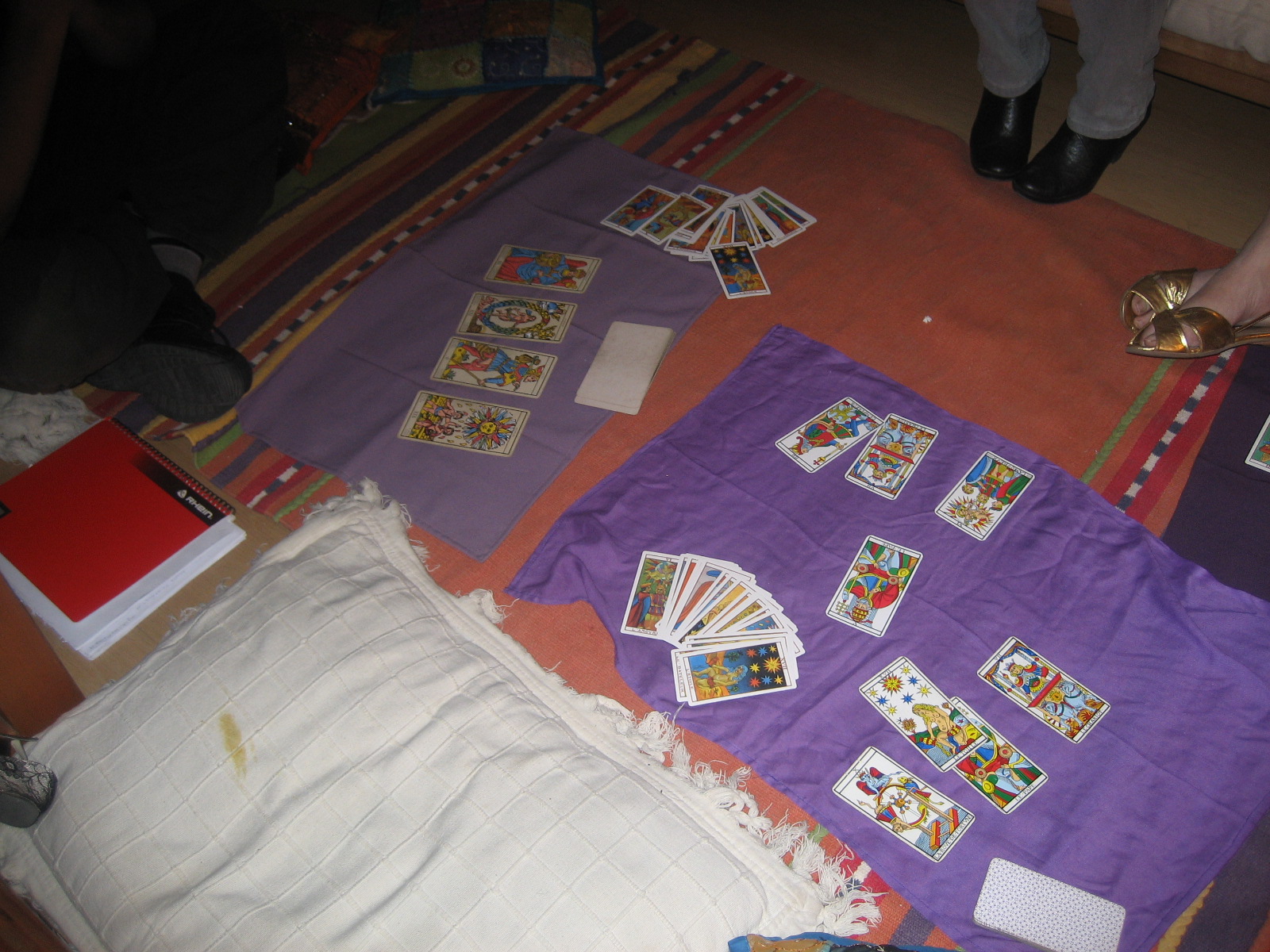This photo captures a dimly lit scene of what appears to be a tarot reading setup, strewn across a light brown wooden floor. The floor is mostly covered with various blankets in different colors and patterns, creating a chaotic yet intriguing arrangement. The most prominent blanket is a large red-orange one with numerous vertical stripes in tan, brown, red, pink, blue, yellow, orange, black, white, yellow, green, blue, and red hues, along with a sizable orange square in the center.

Toward the front right, a purple blanket is spread out with tarot cards placed on it. Another lighter purple blanket is situated vertically near the left-center of the image. A white pillow, or pillow-like object, can be seen on the ground, featuring a stringy edge and a yellow stain on its left end. Adjacent to this pillow lies a stack of notebooks, with the top one being red while the others remain partially obscured.

The photo also includes partial views of three individuals, displaying only their feet—some standing, some sitting—around the setup. Tarot cards are scattered across the various blankets, adding to the mystic and somewhat cluttered ambiance of the scene. The overall dark and poor quality of the photo adds a layer of mystery, leaving much to the imagination.